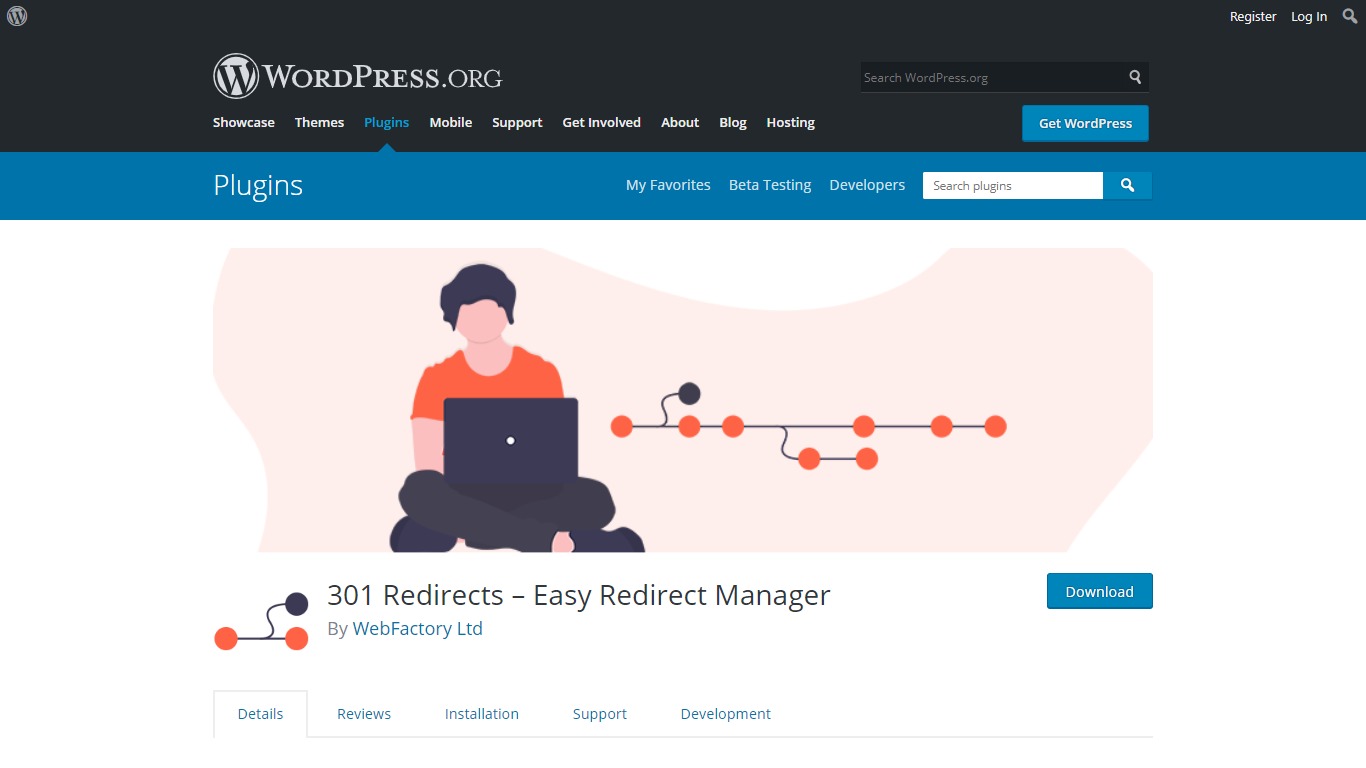This is a detailed caption to describe the screenshot:

---

The screenshot is taken from the top right corner of the WordPress.org website. In the top right corner, there are tabs for "Register," "Log In," and a search icon represented by a small magnifying glass, situated beneath the "WordPress.org" text and its logo, which is a stylized "W" enclosed within a circle with a white outline surrounding it. Below this, there is a navigation bar with nine tabs, each consisting of one or two words: "Showcase," "Themes," "Plugins," "Mobile," "Support," "Get Involved," "About," "Blog," and "Hosting."

In the main window of the screenshot, a central image features an individual wearing a red t-shirt. The person is seated cross-legged on the floor with a laptop resting on their legs, appearing to be engaged in work. The background behind the individual features a creatively designed pink shape.

Beneath this image, there is a text that reads: "301 Redirects - Easy Redirect Manager by Web Factory Ltd." Directly below this text is a blue button with white text that says "Download." Further down, the interface shows an additional five tabs, though their specific titles are not visible in this portion of the screenshot.